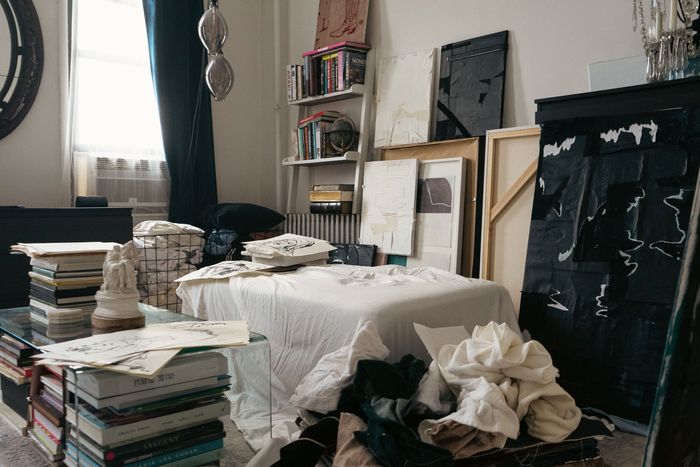The photo showcases a possibly cluttered art studio or artist's office inside a house. The space is filled with various items that suggest creative activity. Central to the image is a clear glass coffee table, heavily laden with books, sketches, and other papers. Below the table, more books are stacked, providing additional storage. Adjacent to this setup is an ottoman, draped with a white sheet, also covered with sketches. The back wall features a window shaded by a dark curtain, flanked by wire hampers filled with fabrics and clothes. 

On the right side of the room, several canvases, some blank and others painted, lean against the wall, hinting at ongoing art projects. Behind the table is a bookshelf, approximately six feet tall, crammed with numerous books and topped with what might be more sketches or a decorative object. The lower part of the bookshelf is partly obstructed by more frames and canvases, further emphasizing the artistic use of the room. Overall, the space appears to be a well-worn and functional area dedicated to artistic endeavors.